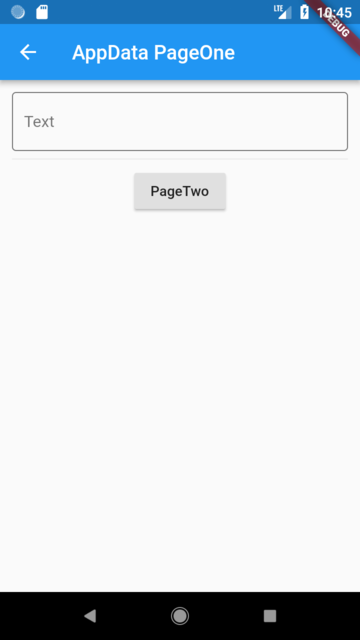The web page displayed is predominantly blue, featuring "App Data Page 1" as its main heading. Below this heading, there is a white text box, and further down, a clickable link labeled "Page 2" is available for navigation. The page is unfamiliar to the observer, leaving them unsure of its specific function. In the top left corner, there are several icons, including one that resembles a uniquely shaped padlock, though its exact nature is uncertain. A dark blue horizontal stripe runs along the very top of the web page, above the usual status icons that indicate battery life and the current time, which reads 10:45. Beneath these status icons, a diagonal brown stripe cuts across the screen, partially obscured, but enough of it is visible to discern the white lettering "BUG," potentially hinting at a word like "debug."